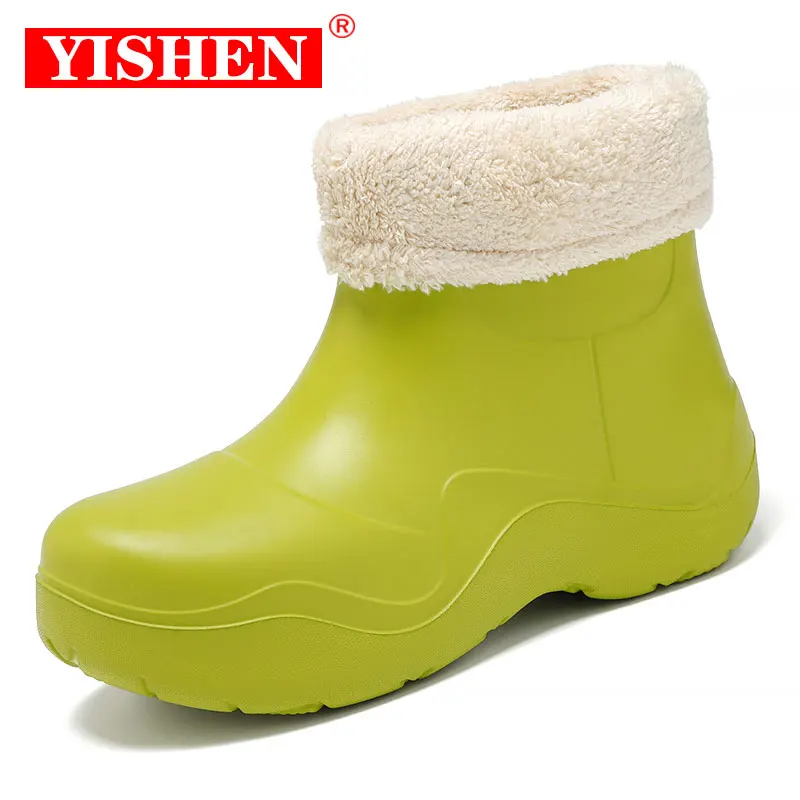This image features a small child's snow boot, approximately ankle height, facing to the left. The boot is crafted from hard rubber and displays a chartreuse color, which is a yellow-green hue with shiny areas at the toe and the top. The exterior rubber appears durable, suitable for snowy conditions. At the top of the boot, there is a folded-down cuff made from a fluffy, smooth white faux fur, providing a cozy touch. The interior of the boot is also lined with this same luxuriant white faux fur, enhancing its warmth and comfort.

Positioned conspicuously on the upper left side of the boot is the brand logo. This is depicted as a red rectangle featuring the brand name "Yishen" in white capital letters (Y-I-S-H-E-N). Accompanying the logo is a small red registered trademark symbol (®) in the upper right-hand corner of the rectangle. A shadow beneath the boot extends straightforwardly down, suggesting it is being viewed under a direct light source. This single, prominently displayed boot effectively highlights the Yishen brand's offering of children's snow boots.